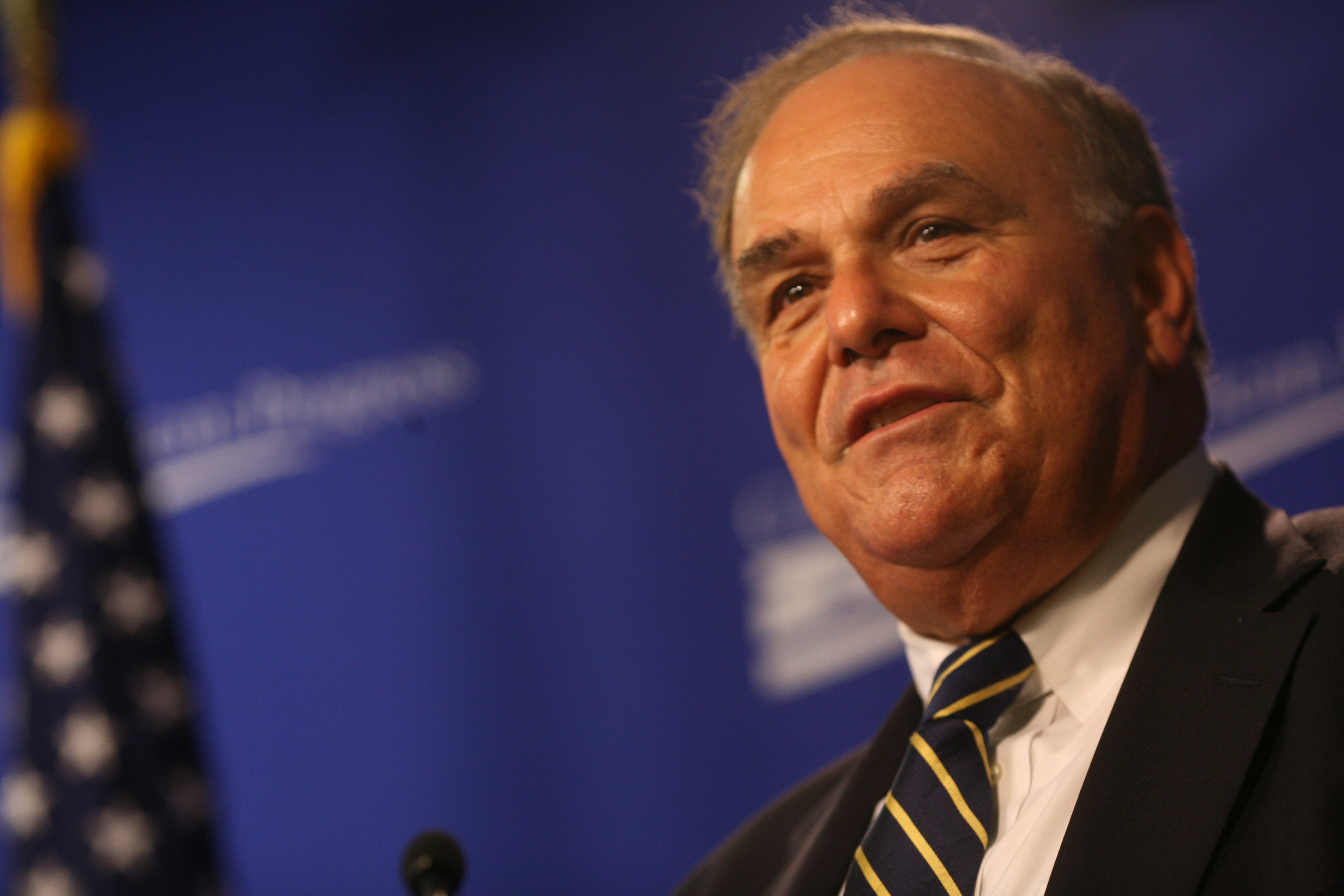The image depicts a politician standing at a podium, speaking to an unseen crowd. He has short, graying hair and is smiling warmly, his expressive, thick eyebrows contributing to a friendly demeanor. He is dressed in a black suit jacket, a white collared shirt, and a navy blue and gold-striped tie. A black microphone is positioned in front of him. The backdrop features a prominent dark blue curtain with blurry white writing, adding a formal atmosphere to the scene. To the left side of the image, partly obscured, is the iconic American flag with white stars on a blue field and a yellow sash at the top. The politician's positioning to the right of the frame and his attire together with the setting suggest he is addressing an important gathering or event.